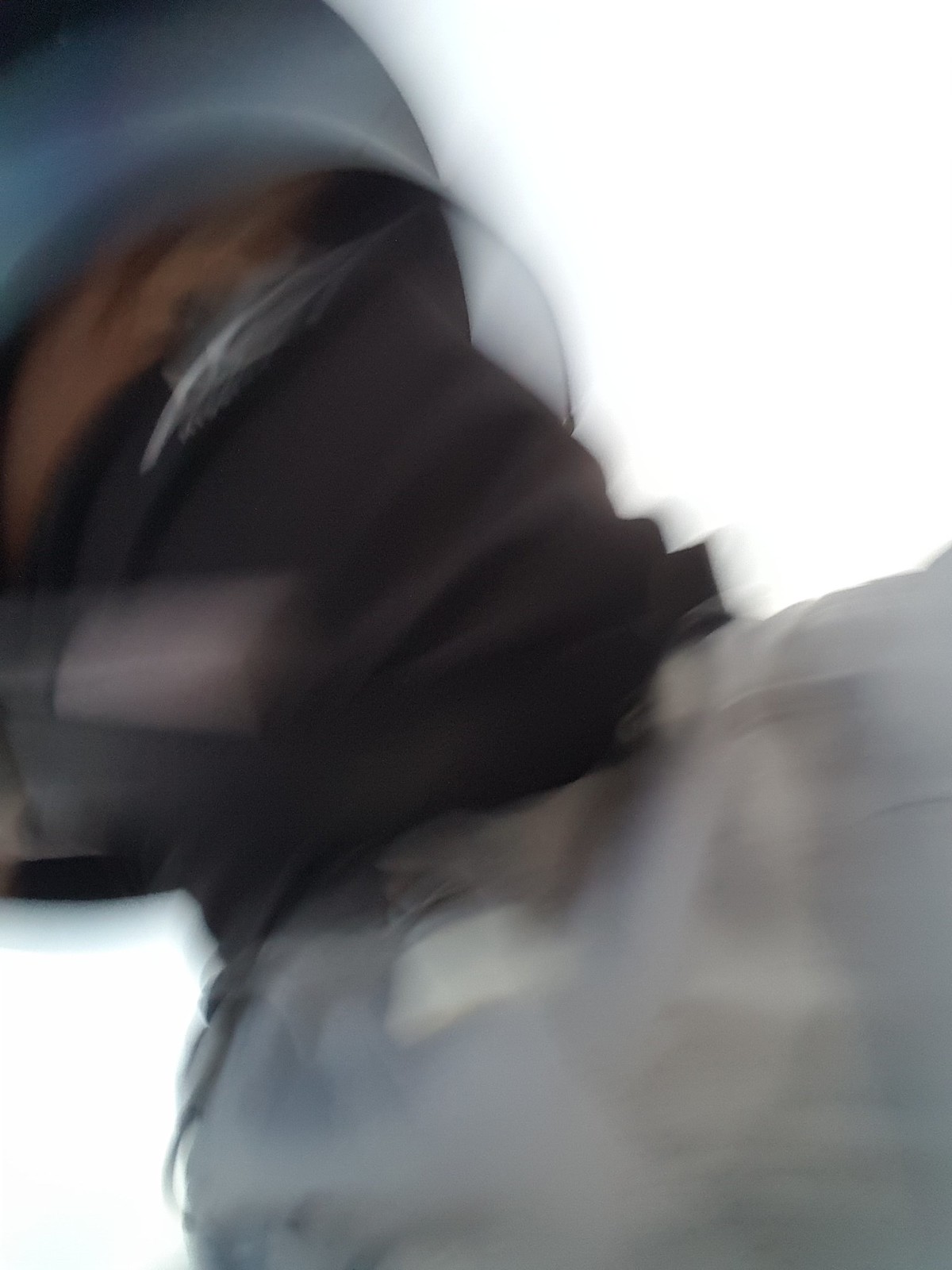This blurry photograph depicts what appears to be a person, whose precise details are obscured by motion. The figure seems to be wearing a black face shield, a possible military or motorcycle helmet with a blue top, and potentially a patterned uniform, indicating a military context. Around the head area, there can be seen a foamy white ring, with what might be headphones near the ears. The image might include round eyebrows and hints at the presence of clear plastic. The bottom corner and nearly the entire lower portion of the picture are dominated by a big gray blob. The overall impression is one of a heavily obscured figure, possibly in a military or specialized uniform, captured in a moment of swift motion or blur.